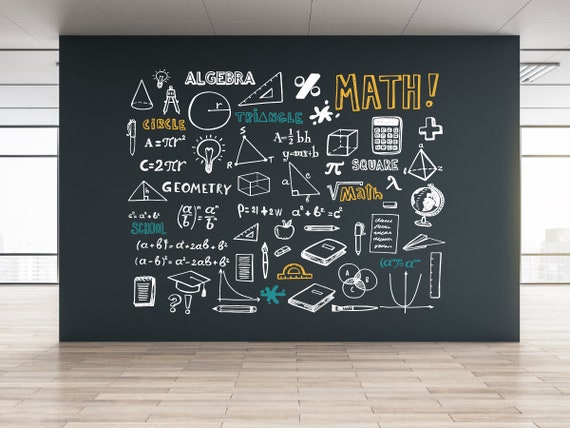This image captures a lively and whimsical floor-to-ceiling feature wall in what appears to be an office or school setting. The wall, painted entirely with black chalkboard paint, showcases an artistic array of handwritten mathematical terms and symbols in various vibrant colors, including blue, white, black, orange, and a distinctive goldish yellow for the word "MATH." The design intricately spans from the light stone floor to the ceiling, integrating a plethora of math-related graphics and words such as algebra, geometry, the word "square," and several math equations. The wall is adorned with illustrations of mathematical items like a radius symbol, square roots, books, a pen, calculators, a globe, and a graduation cap. Additional shapes such as a cone, cube, and pyramid are also depicted. The overall atmosphere is enhanced by elements hinting at a classroom environment, including ceiling tiles, fluorescent lighting, and possibly a window in the background, which all highlight the educational significance of the mural.